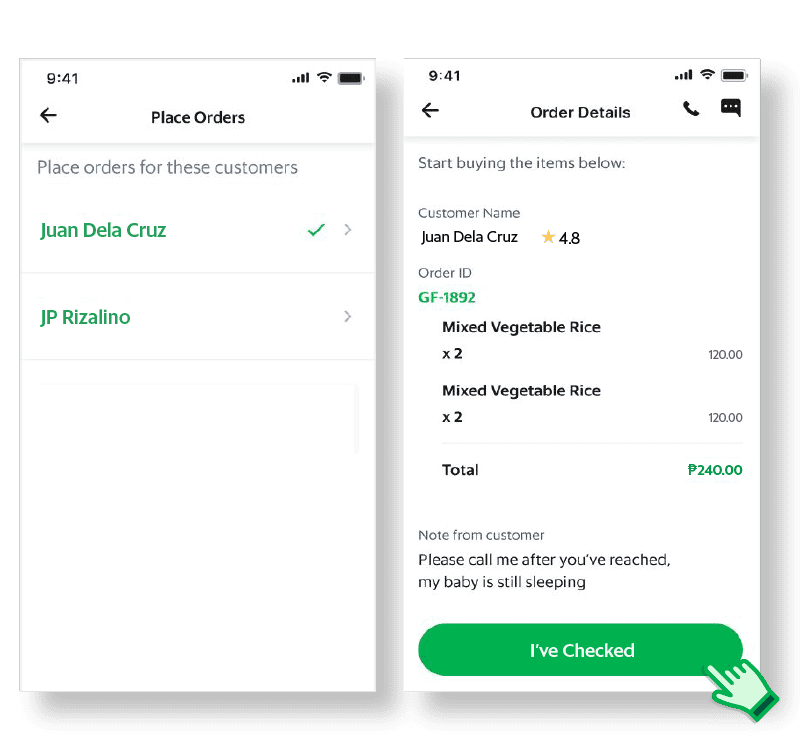This image is a composite screenshot from a smartphone, illustrating a buying or order process, possibly for a delivery service like Instacart or UberEats. Both screenshots display a time of 9:41 and show similar battery levels at approximately 98%.

On the left screenshot, the screen is titled "Place Orders." Below, instructions prompt the user to place orders for two customers, highlighted in two separate lines: Juan de la Cruz, marked with a checkmark indicating completion, and JP Rizzolino, without a checkmark suggesting the order is pending.

The right screenshot appears to be the subsequent step in the process for Juan de la Cruz. The screen is headed "Start buying the items below," listing Juan de la Cruz with a customer rating of 4.8 out of 5. Below, the ordered items are specified: two mixed vegetable rice portions in two separate orders.

This detailed depiction shows a step-by-step order process, likely involving direct interaction at a restaurant or store to fulfill customer orders.